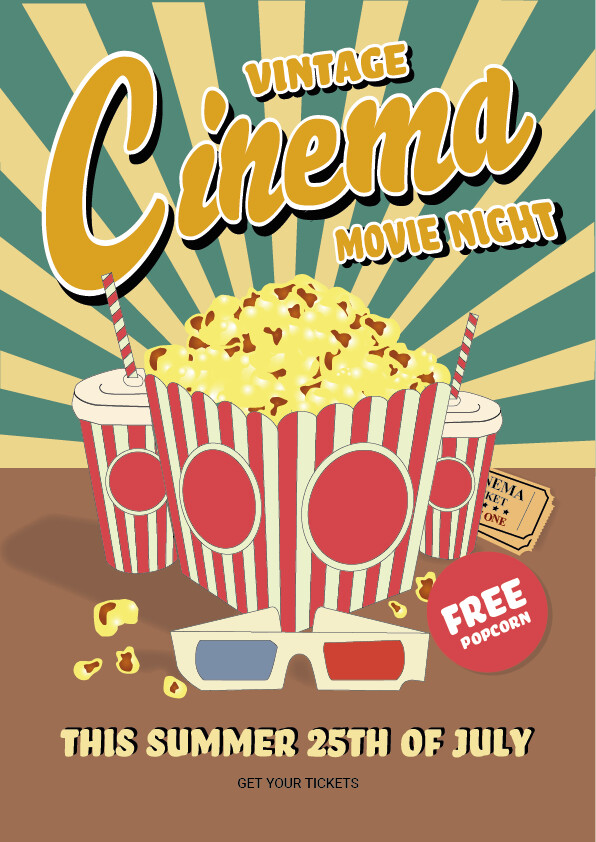The advertisement poster boasts a vintage, retro style, with artistic computer-generated graphics designed to replicate an old movie poster. The prominent text in varying shades of yellow reads "Vintage Cinema Movie Night" at the top, with "Cinema" in large cursive font, and "Vintage" and "Movie Night" in regular font. Toward the bottom, it reads "This Summer, 25th of July" and "Get Your Tickets" in black font.

The background features sunbeam stripes in yellow and bluish-green, radiating outward and creating a nostalgic ambiance. Positioned centrally on the poster is a classic red and white striped popcorn box, showcasing yellow popcorn with some blackened kernels. This is flanked by two matching red and white striped soda cups, complete with lids and black straws. In front of the popcorn, there are 3D glasses with one lens in red and the other in blue, enhancing the retro appeal.

Additional elements include two halves of cinema tickets and text indicating "Free Popcorn" in white font, accompanied by a few scattered popcorn kernels. This visually captivating and stylized poster effectively conveys the event's theme and details, combining nostalgic imagery with essential information for an inviting and memorable Vintage Cinema Movie Night.